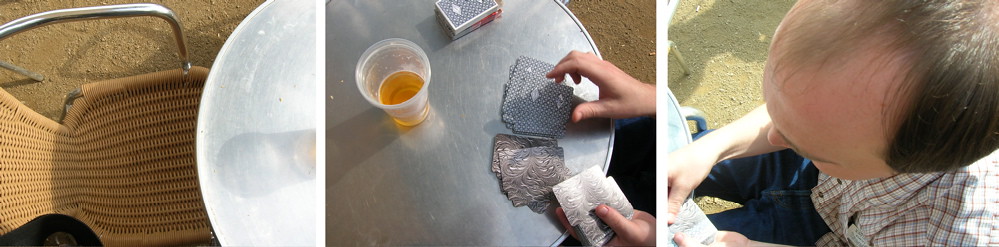The image is a triptych of three vibrant photographs centered around a table. 

In the first photograph on the left, a cork-braided chair takes the spotlight. The chair, woven in shades of brown, is paired with sleek silver arms. It stands on a brown cement floor and is pulled up to a round table with a shiny metal surface, of which only a small portion is visible.

In the center photograph, more of the table is revealed. Atop the polished surface sits a plastic cup filled with a pale golden liquid, likely beer. Nearby, a deck of playing cards is scattered, and the box is visible. Two human hands are caught in the middle of shuffling the cards, enveloping the scene in an air of anticipation.

The rightmost photograph shifts focus to a man seen from above. His thinning brown hair and receding hairline are conspicuous. He is dressed casually in a plaid shirt and blue jeans. The man's hands grasp the playing cards, while the stone floor beneath him subtly contrasts with the rest of the tableau.